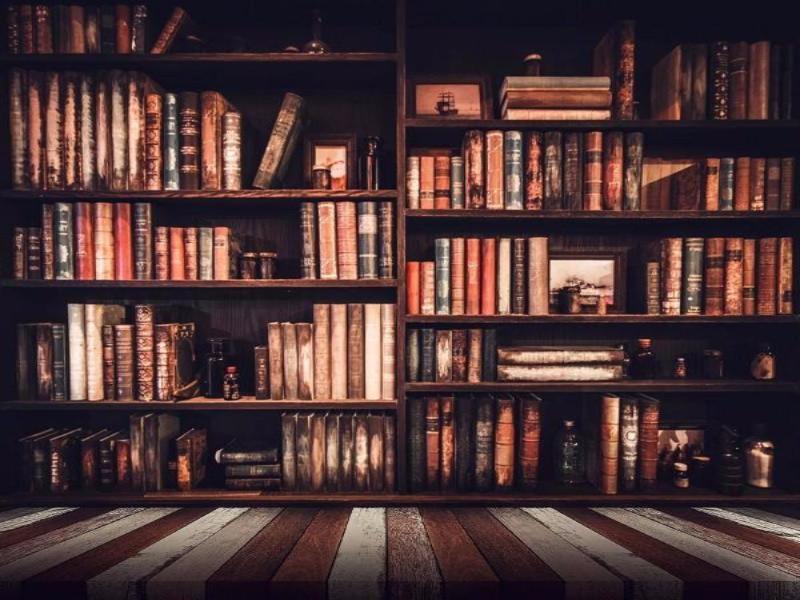The image captures a dimly lit, richly toned study within a house, featuring an expansive, dark brown wooden bookcase that spans the entire visible height and width of the wall. The bookcase is densely packed with weathered, antique books in various shades of brown, blue, tan, beige, and occasional reds, each exuding a well-used, vintage charm. The shelves are arranged in a five-by-five grid, with books both vertically aligned and some horizontally stacked in groups of three. Interspersed among the books are various decorative items such as vases, bottles, and framed pictures of ships and memorable moments, adding depth and texture to the scene. The floor consists of alternating wooden planks in lighter and darker hues, complementing the bookcase's rustic aesthetic. The overall ambiance suggests a professional photo shoot capturing the nostalgic and scholarly atmosphere of a well-loved, antiquated library.